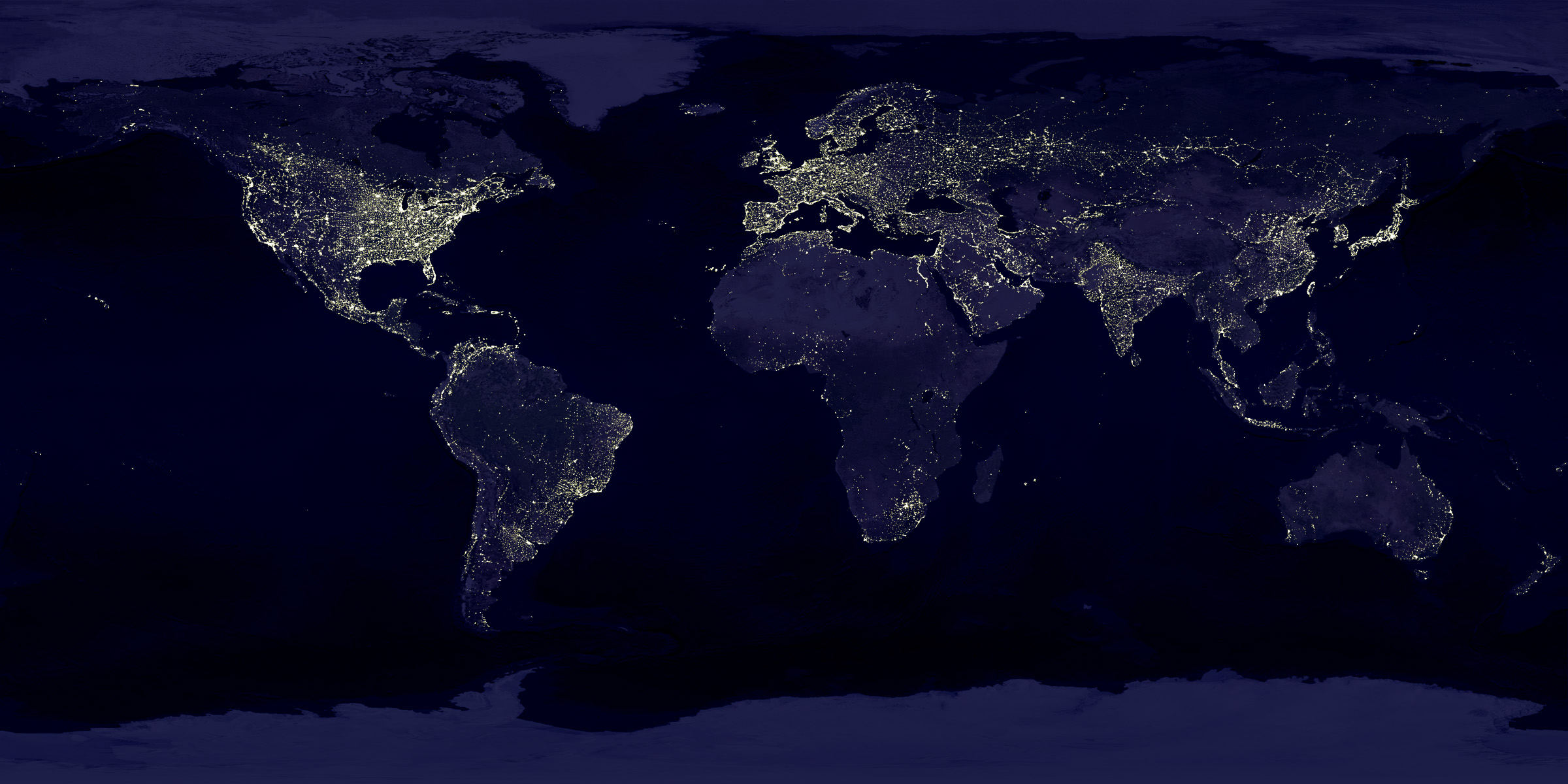This image is a detailed, digital artist’s rendering of a world map displayed as if laid flat on paper. The background is a deep, midnight blue, representing nighttime, with each continent depicted in a lighter shade of blue. Some areas, particularly parts of North America, are highlighted in a yellowish hue, indicating more densely populated regions. The map illustrates light pollution, showing where cities are brightened by human activity. The eastern United States and Europe, particularly the UK, France, and surrounding areas, exhibit the highest concentrations of light. Other regions such as South Asia, the Middle East, Japan, and parts of China also display significant light clusters. In contrast, continents like Africa and Australia show fewer lights, mostly concentrated along their coastlines. The map includes all continents, emphasizing the global distribution of light pollution, with Antarctica also depicted in this nightscape.